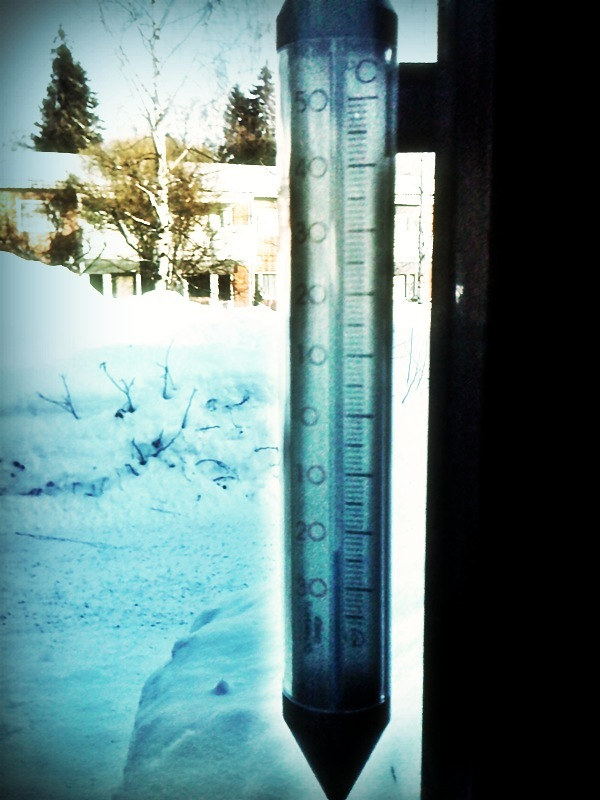The image features an outdoor scene centered around a thermometer. The thermometer is clear, with a subtle bluish tinge, but the exact temperature it shows is indiscernible. Behind the thermometer, a vast snow-covered landscape unfolds. To the left, a significant amount of snow appears with a bluish tint, leading to a tall snowbank. Further back, a large white house stands prominently, surrounded by snowfall. In front of the house, a tall, thin tree with numerous branches rises, displaying either foliage on its lower branches or possibly another tree behind it. In the distant background, evergreen trees are visible, adding depth and contrast to the snowy scene. To the right of the image, a portion of the frame is occupied by a black area with a small white squiggle, making it seem like a drawing rather than a photograph.